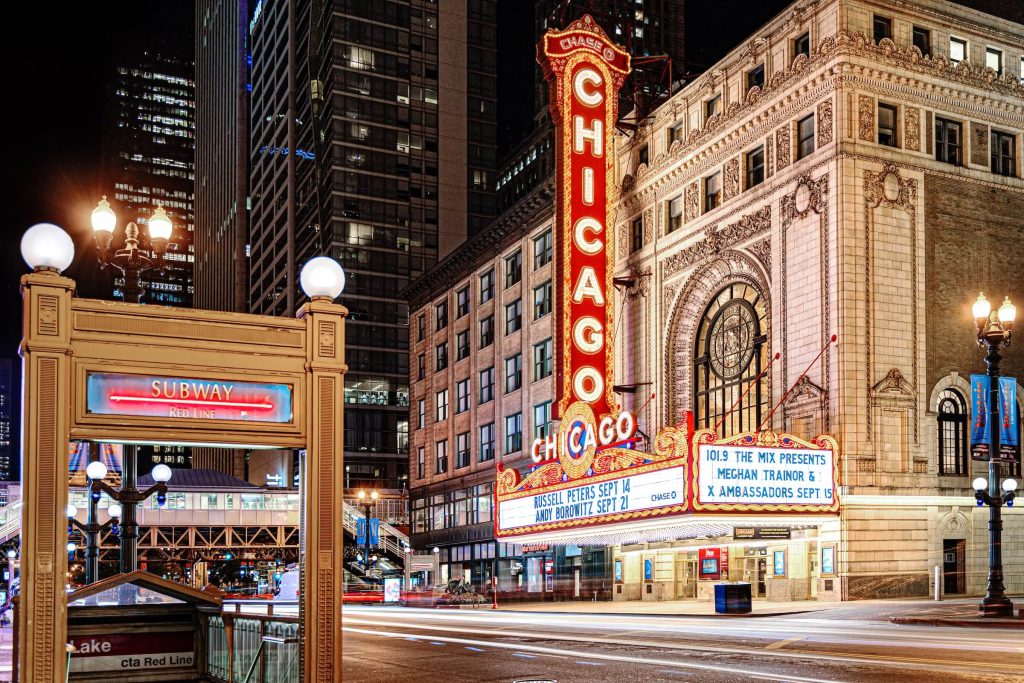The photograph captures a nighttime scene in downtown Chicago, vividly illuminated against the dark sky. Dominating the right half of the image is the historic Chicago Theater, a notable landmark characterized by its ornate architecture in browns, reds, and golds. The eye-catching vertical sign prominently displays the word "Chicago" in white letters with a red background and a yellow outline. Below this, marquee advertisements announce upcoming events: "Russell Peters September 14th," "Andy Borowitz September 21st," and "101.9 The Mix presents Meghan Trainor and X Ambassadors September 15th." The theater's entrance features ticket booths beneath the illuminated marquee. To the left, a Subway sign marks the entrance to the Lake Street Tram, while blurred skyscrapers loom in the background, their few lights adding depth to the scene. The empty street suggests the photograph was taken very late at night or early in the morning, adding an eerie tranquility to this vibrant urban snapshot.